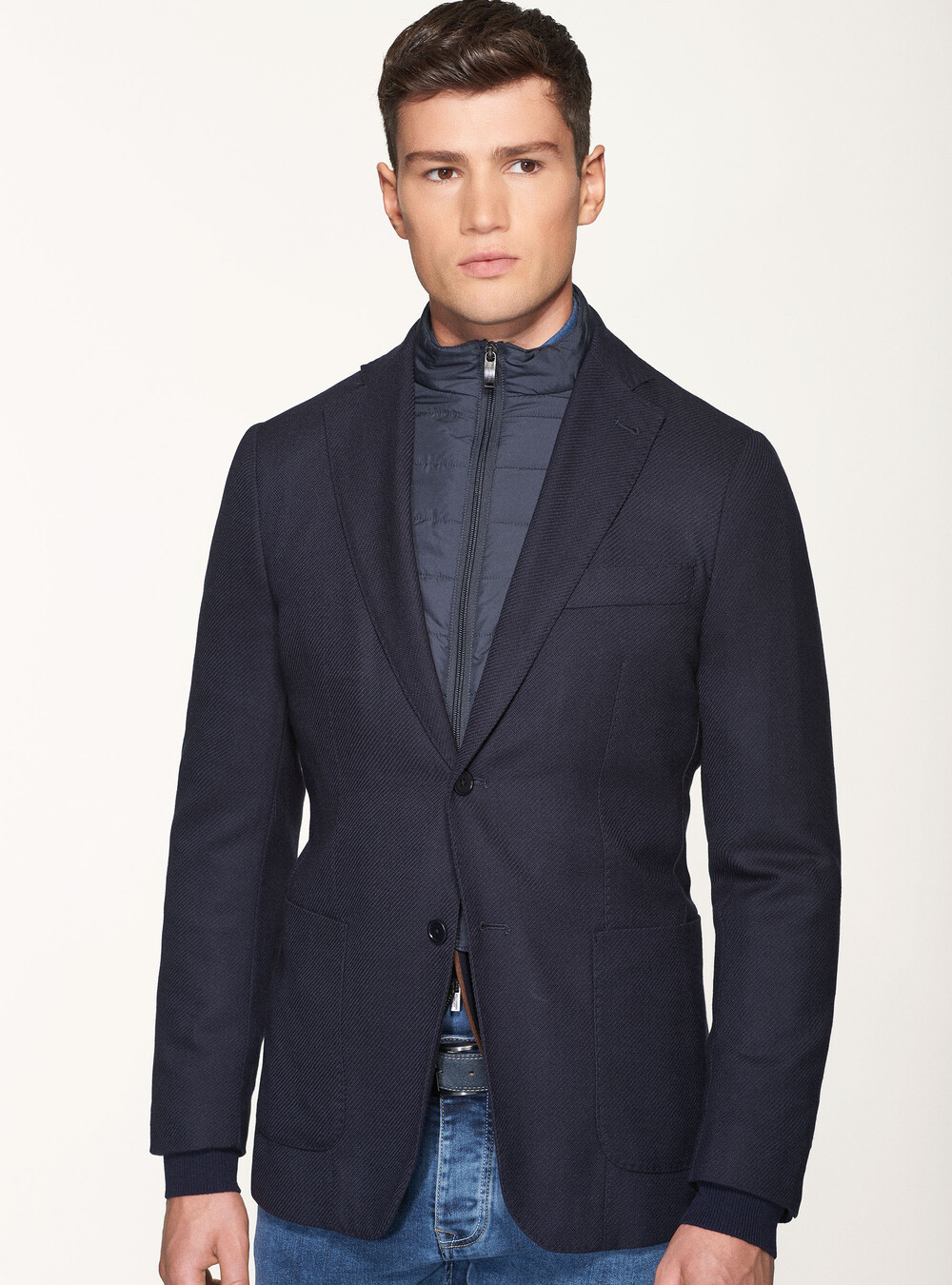The image is a detailed, photographic portrait of a clean-shaven Hispanic man in his 20s, set against a light gray, whitish background, likely indoors. The man has short, wavy dark hair, which is slightly longer on top and neatly styled off his forehead. His head is subtly tilted from right to left, and he gazes slightly away from the camera, adding to the candid and introspective feel of the photo.

He is dressed in a shiny, dark gray sports jacket, with the top button fastened and the second button left undone. Beneath the jacket, he wears a zippered gray vest, hinting at an athleisure style, which fits snugly around his torso. His attire includes blue jeans secured by a gray belt with a silver buckle, complementing his overall modern and stylish look.

The image captures him from head to just below his crotch, with his arms resting naturally at his sides. You can see the sleeve of the vest extending slightly beyond the jacket's sleeve near his wrist. The right hand shows more prominently, with his thumb and fingers partially visible, while the left hand fades out of view. The man's poised stance and fashionable attire suggest he might be a model, possibly highlighting the clothing's details in this sophisticated and polished photograph.